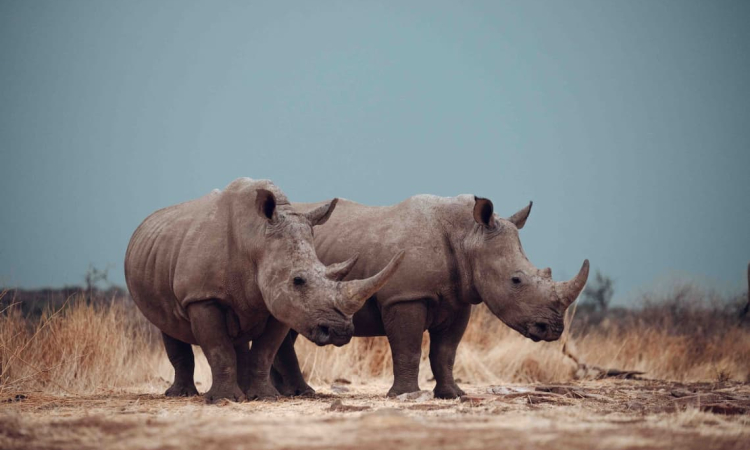In this detailed image, we see two wild rhinoceroses standing side by side in the center of a vast savanna. They both face towards the right. The rhino on the left has slightly longer horns, while the rhino on the right features distinct white spots on its head and gray pigmentation. Their thick legs and robust build are evident. The landscape around them is characterized by dirt and tall yellow grasses, typical of a savanna, with some broken sticks scattered behind the rhinos. In the background, some trees are visible, and the sky is a bluish-gray, creating a serene and natural setting. There is no text in the image to distract from this captivating scene of wildlife.